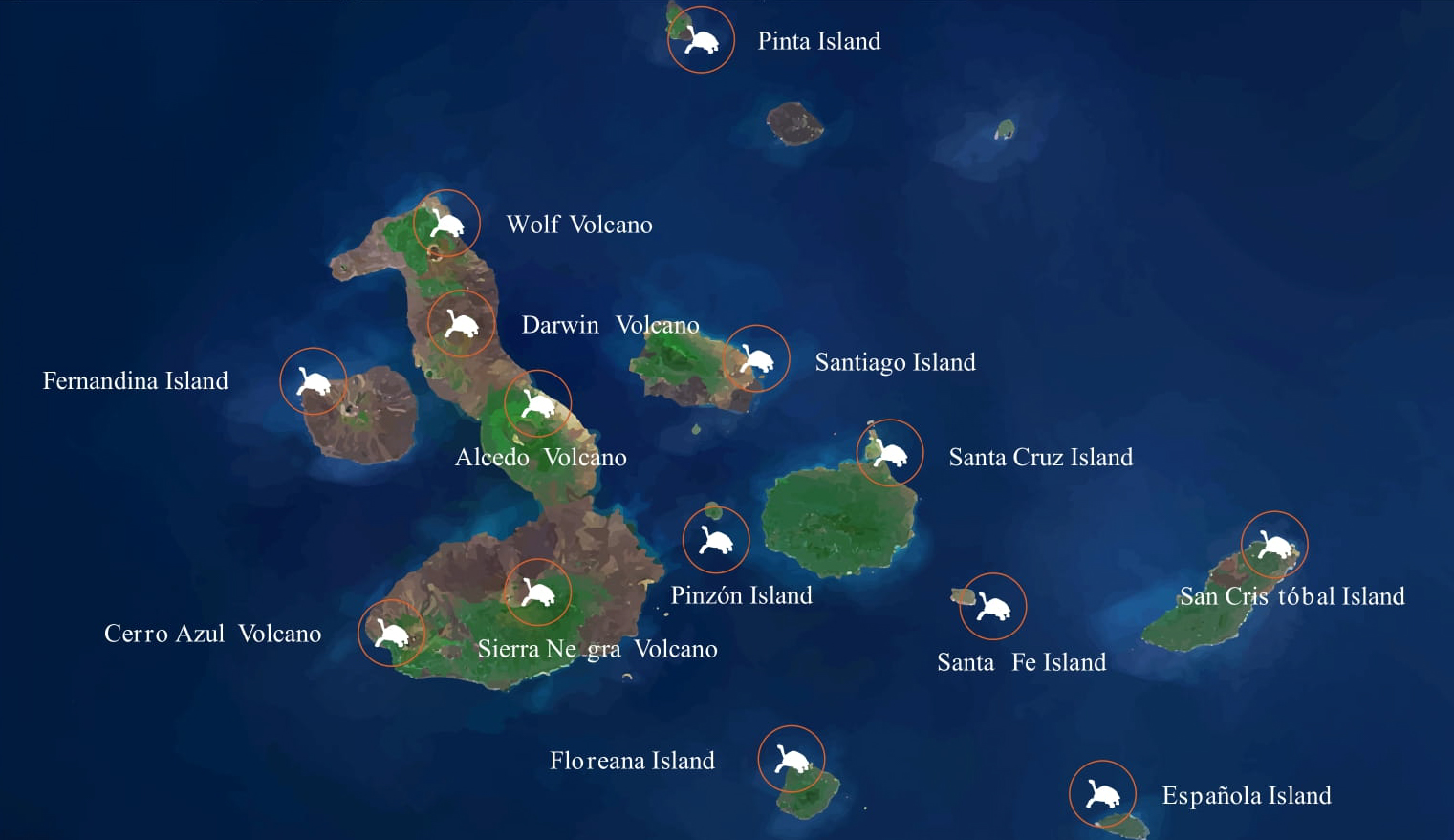This is a detailed color map illustrating a cluster of islands set against a sea of dark and lighter blue patches. At the top of the map is Pinta Island, depicted as a small brown island. The map features several medium-sized and small islands, among which are Fernandina Island, Santiago Island, Santa Cruz Island, Santa Fe Island, San Cristobal Island, and Española Island. Among the notable geographical features are numerous volcanoes labeled with white print, including Wolf Volcano, Darwin Volcano, Alcido Volcano, Cerro Azul, and Sierra Negra. Additionally, the map displays many icons resembling leaping cats.